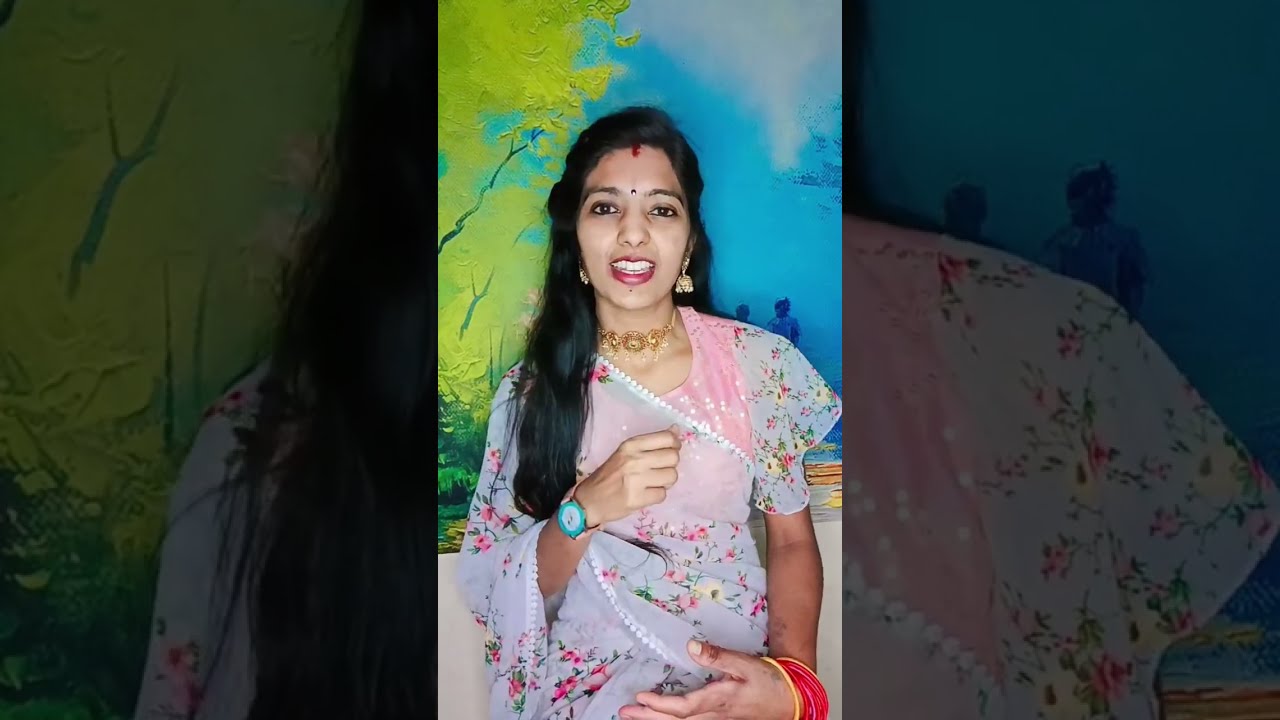The image is a three-paneled photograph with the left and right panels darkened and showing close-up versions of the brighter center image, which is the focal point. The center panel features a woman of Indian descent standing before a painted backdrop that depicts blue skies with cloud shapes, tree branches with yellow leaves, and possibly a stone path with people painted behind her left shoulder. The woman has long, dark hair adorned with a red bindi on her forehead and a rhinestone between her eyebrows. She is smiling and wearing bright red lipstick. Her attire includes a translucent floral shawl over a pink top, which has pink flowers with green branches embroidered on it. She accessorizes with two large gold earrings, a tight gold choker necklace, several bracelets on her left wrist, and a blue-rimmed wristwatch with a white face and pink bands on her right wrist. The overall ambiance of the photo is enriched by the intricate details of both her attire and the artistic background.